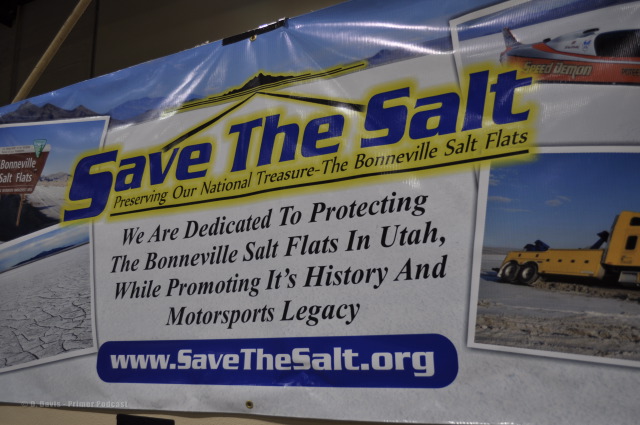The banner promoting the "Save the Salt" initiative features a prominent title in large blue letters at the top, stating "Save the Salt." This is followed by the tagline, "Preserving our national treasure, the Bonneville Salt Flats," in black, underlined font. The banner has a white background with centered black text that says, "We are dedicated to protecting the Bonneville Salt Flats in Utah, while promoting its history and motorsports legacy." At the bottom, a blue oval with white lettering provides the website, "www.savethesalt.org." The background includes a scenic image of the Salt Flats with hills under a blue sky. On the right side of the banner, there are partial images of a yellow construction vehicle and a car labeled "Speed Demon."